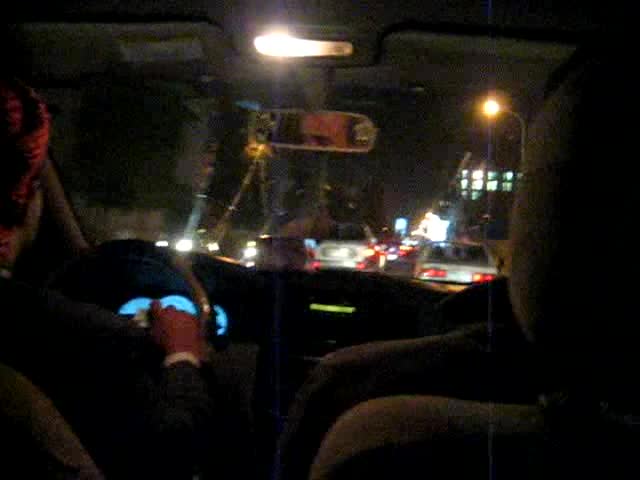The image depicts the interior of a car at night, with the vehicle's dashboard illuminated. The car has a left-hand drive, indicating it might be from a European country. The driver, who appears to be of European descent, is dressed formally in a long-sleeved coat with a white polo shirt underneath. He is wearing a red turban-like headwear, although the specific type of hat is unclear. The driver’s hands are firmly on the steering wheel. Sitting to his right in the passenger seat is an individual wearing a dark gray coat, but further details about this passenger are not discernible. The scene outside the car shows heavy traffic in the city, suggesting slow movement or a complete standstill. There is a counter flow of traffic on the left side of the vehicle. The sky outside is pitch black, indicating that the photo was likely taken between 9 p.m. and 10 p.m.